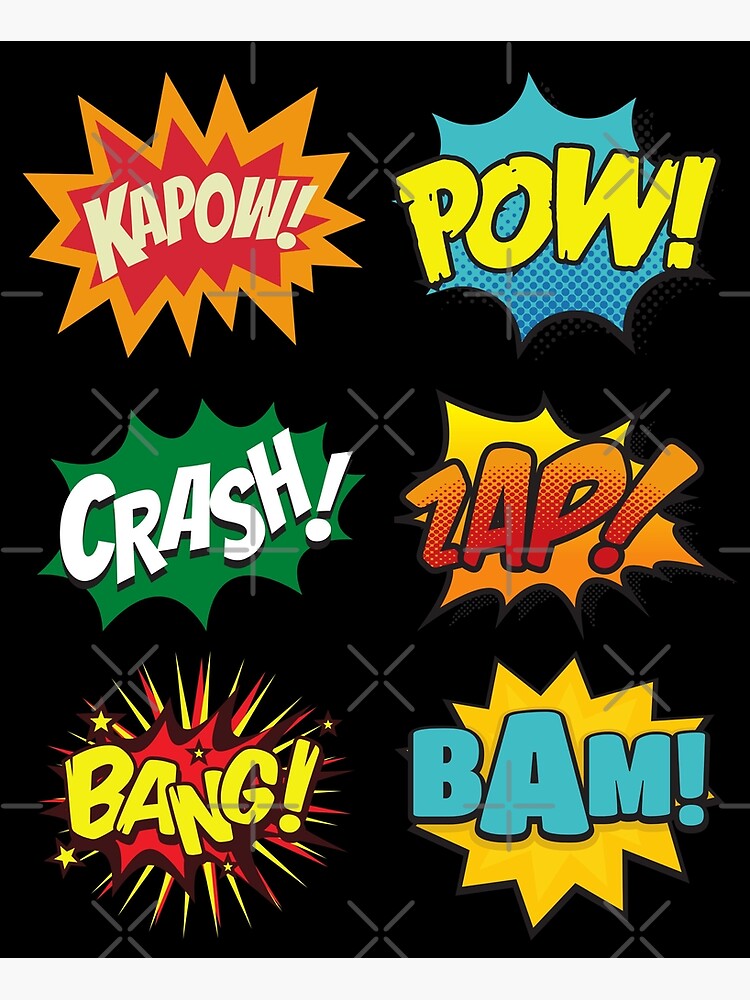The image is a vivid, comic book-style graphic featuring six distinct sound effect bubbles arranged in two columns against a black background. The left column includes:

1. "Kapow!" in bold white letters, backed by a jagged red and orange explosion.
2. "Crash!" in white font, set against a bright green scalloped background.
3. "Bang!" in yellow letters with a dynamic red and yellow scalloped background, accompanied by yellow stars and rays.

The right column features:

1. "Pow!" in bright yellow letters on a blue scalloped-edge bubble.
2. "Zap!" in red-orange gradient letters, with an orange and yellow explosion behind it.
3. "Bam!" in light blue letters against a yellow jagged background.

Each bubble has a distinct and colorful design, evoking the classic action and energy of comic book sound effects. The high contrast and sharp details suggest this might be a graphic design template. The overall look is vibrant and dynamic, capturing the essence of comic book excitement with its explosive typography and bold colors.